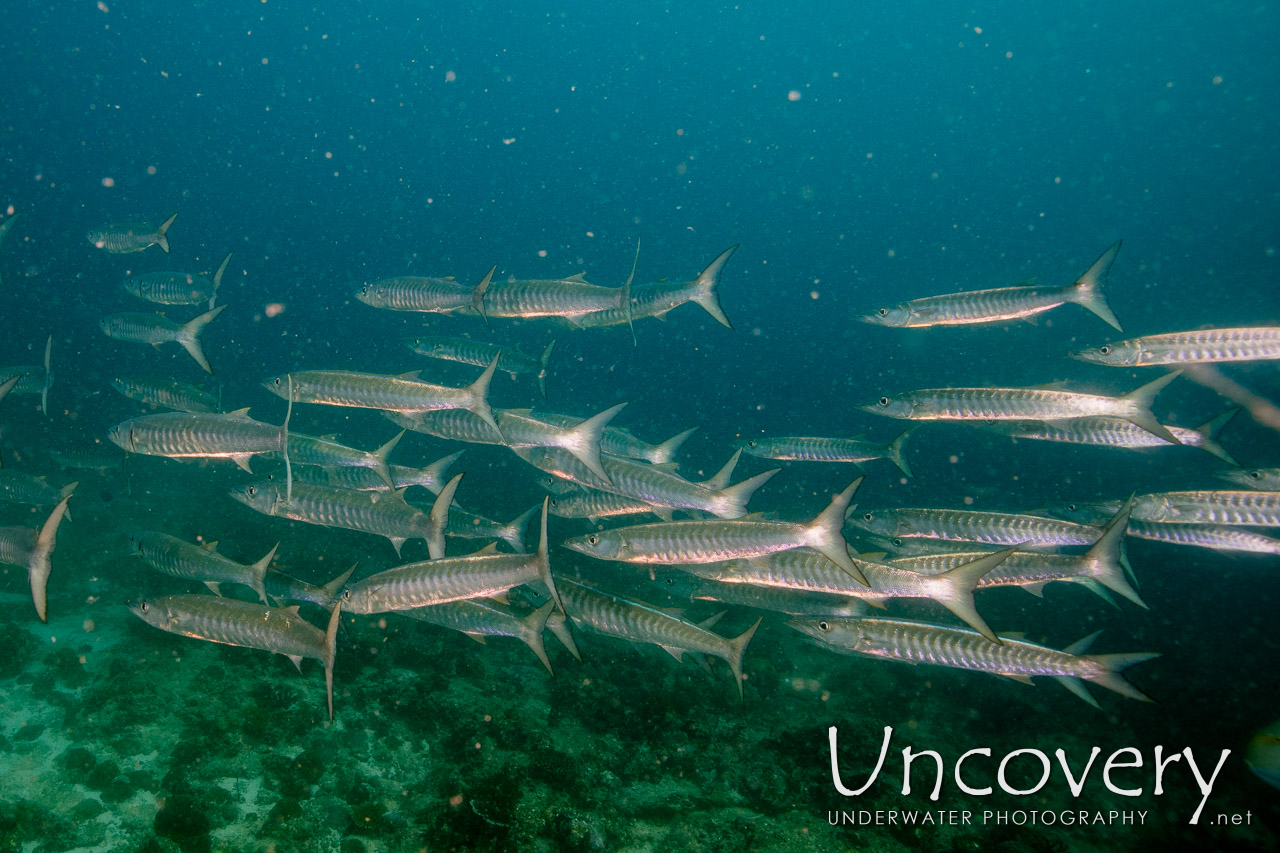The horizontally aligned rectangular image captures an underwater scene with a large school of narrow, elongated fish, each with a silver-gray upper body and a tan or orange-tinged underside. The fish, all of the same species, swarm densely toward the left side of the image. The top half of the background showcases a dark blue hue peppered with light gray or white specks, creating a textured, almost grainy visual effect. The bottom half displays the ocean floor, where sand mixes with hints of plant life, giving off a forest green appearance reminiscent of moss. In the lower right corner, the text "UNCOVERY" is prominently displayed in large white letters, with "underwater photography dot net" in smaller, uppercase white print beneath it.